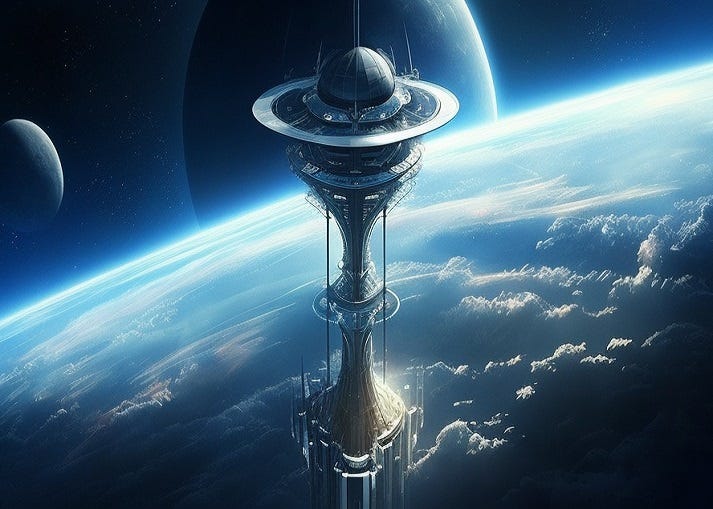The image portrays a highly detailed, AI-generated depiction of outer space, featuring a prominent space station amidst a complex celestial panorama. The central structure is a tall, narrow tower with a round dome at its apex, tapering down through several rings to a wider base, reminiscent of a futuristic space needle. Silver-lit on the sun-facing side and shadowed on the other, the station is adorned with wires or antennae extending from its top. In the background, two planets are visible: one large and prominently circular, and a smaller one on the left. The curvature of another planet's atmosphere is seen slanting upwards from left to right, dotted with wispy, white clouds. Behind this, the dark silhouette of a distant moon contrasts with a lighter crescent on its right side, and another similarly lit moon is positioned towards the outer left edge of the image. The dark expanse of space provides a striking backdrop to this intricate cosmic scene.